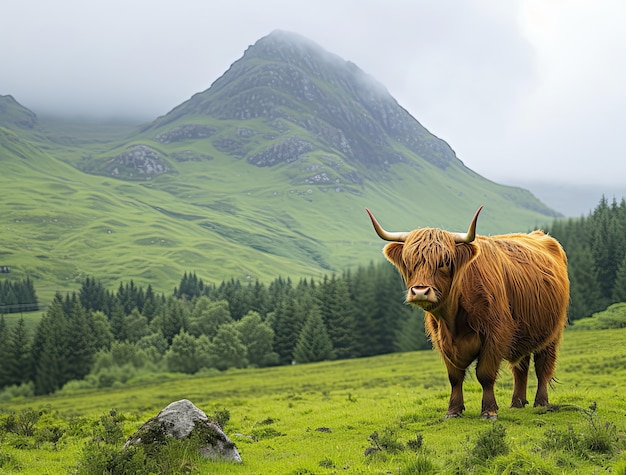The illustration depicts a serene outdoor setting featuring a longhorn steer with a rich, brown coat standing on a grassy surface towards the right-hand side of the image. The animal, which has two prominent horns and hair partially covering its eyes, faces forward toward the viewer. To its left, a gray boulder rests on the ground, adding to the natural ambiance. Behind the steer, a line of fir or pine trees stretches from left to right, leading up towards a large, green, and craggy mountain in the background. The mountain is enveloped in a smoky, misty sky, with sparse clouds that create a sense of a foggy, overcast day. The scene exudes the tranquil beauty of nature, highlighting the harmonious coexistence of wildlife and landscape.